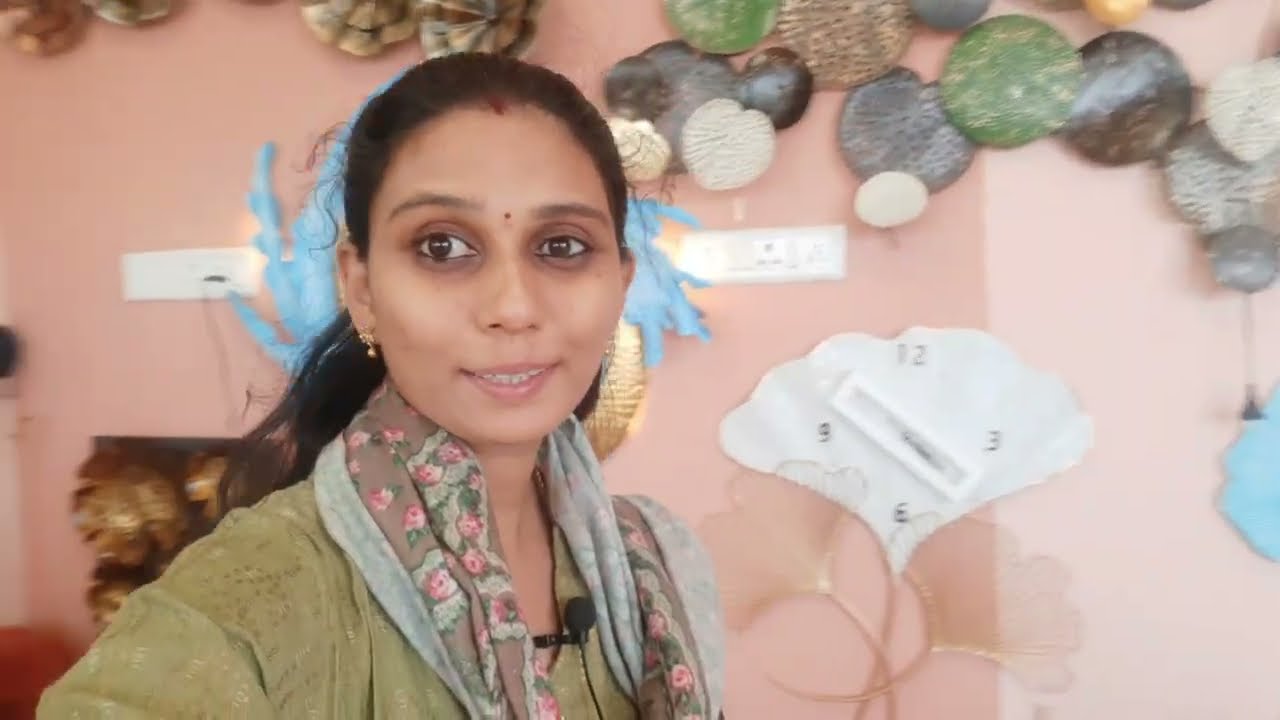This is a detailed landscape photograph of a Middle Eastern woman wearing a green silk blouse paired with a floral scarf adorned with pink, green, and brown designs. She has her hair pulled back into a ponytail and sports henna dye in a line on the middle part of her scalp, including a small maroon bindi dot and another maroon dot between her eyebrows. Her complexion is accentuated by small gold earrings and a warm, open smile that reveals a bit of her teeth. A small microphone is pinned to her collar, indicating she might be speaking or presenting. The backdrop is a peach-colored wall adorned with ornate metal sculptures including textured, circular multicolored plates connected together and a unique white fan-shaped piece numbered 12, 3, 6, and 9. The vibrant artwork in the background, with hues of green, brown, blue, and white, is slightly blurred to emphasize the woman, who is the central focus of the photograph. She stands confidently, left of center, bringing a sense of grace and charm to the composition.